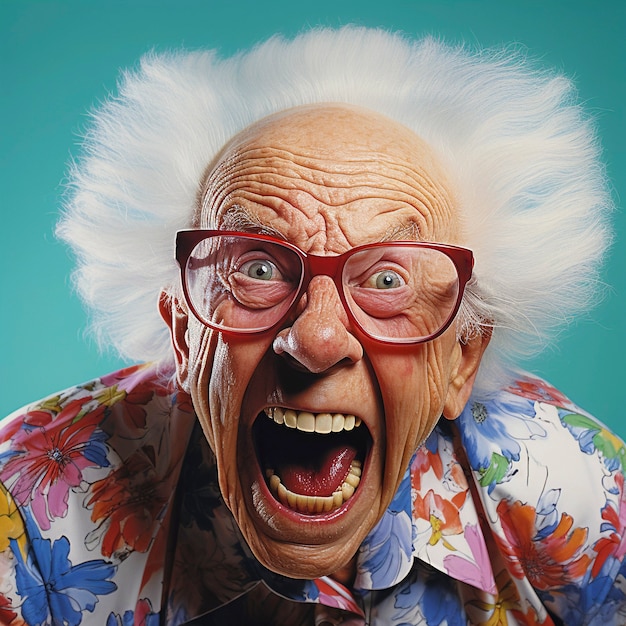The image is a highly detailed, full-color digital print, seemingly AI-generated, depicting an older man in a portrait style. The man is centered in the vertically rectangular frame, staring straight at the viewer with an exaggerated expression of open-mouthed yelling. His face, marked by a receding hairline and deep wrinkles, is adorned with thick red-framed bifocal glasses. His disheveled white hair sticks out wildly, reminiscent of Albert Einstein, creating a halo-like effect around his head. The man wears a vibrant floral Hawaiian shirt featuring colors such as white, blue, red, green, and pink. The background is a cool teal or blue-green color, contrasting with the lively hues of his shirt. Overall, the visual juxtaposition of his cheerful attire and intense expression adds a humorous and surreal touch to the image.